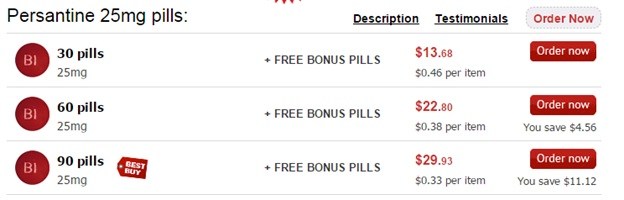The image features a long rectangular layout. At the very top center, there are four arrow-like symbols, suggesting that something might have been cut off from above. Directly beneath these symbols, in black font, it reads "Percentine, 25mg pills." To the right, still in black text, the words "Description" and "Testimonials" are prominently displayed and underlined.

Below this, there is a noticeable rectangular button with red text on a light gray background reading "Order Now." 

Further down, the layout is organized into three distinct lines, each containing a red circle with a white capital "B" next to what appears to be a lowercase "l." The lines detail three different pill quantities: "30 pills, 25mg," "60 pills, 25mg," and "90 pills, 25mg." To the right of the "90 pills" line, there's a small red price tag icon labeled "Best Buy." 

Each line also includes a note about bonus pills added for free. The prices for each quantity are listed as follows:
- 30 pills for $13.68 (46 cents per pill)
- 60 pills for $22.80 (38 cents per pill)
- 90 pills for $29.93 (33 cents per pill)

Alongside each option, there's a red "Order Now" button. Below the "Order Now" button for the 60-pill option, it indicates a savings of $4.56, while the 90-pill option indicates a savings of $11.12.